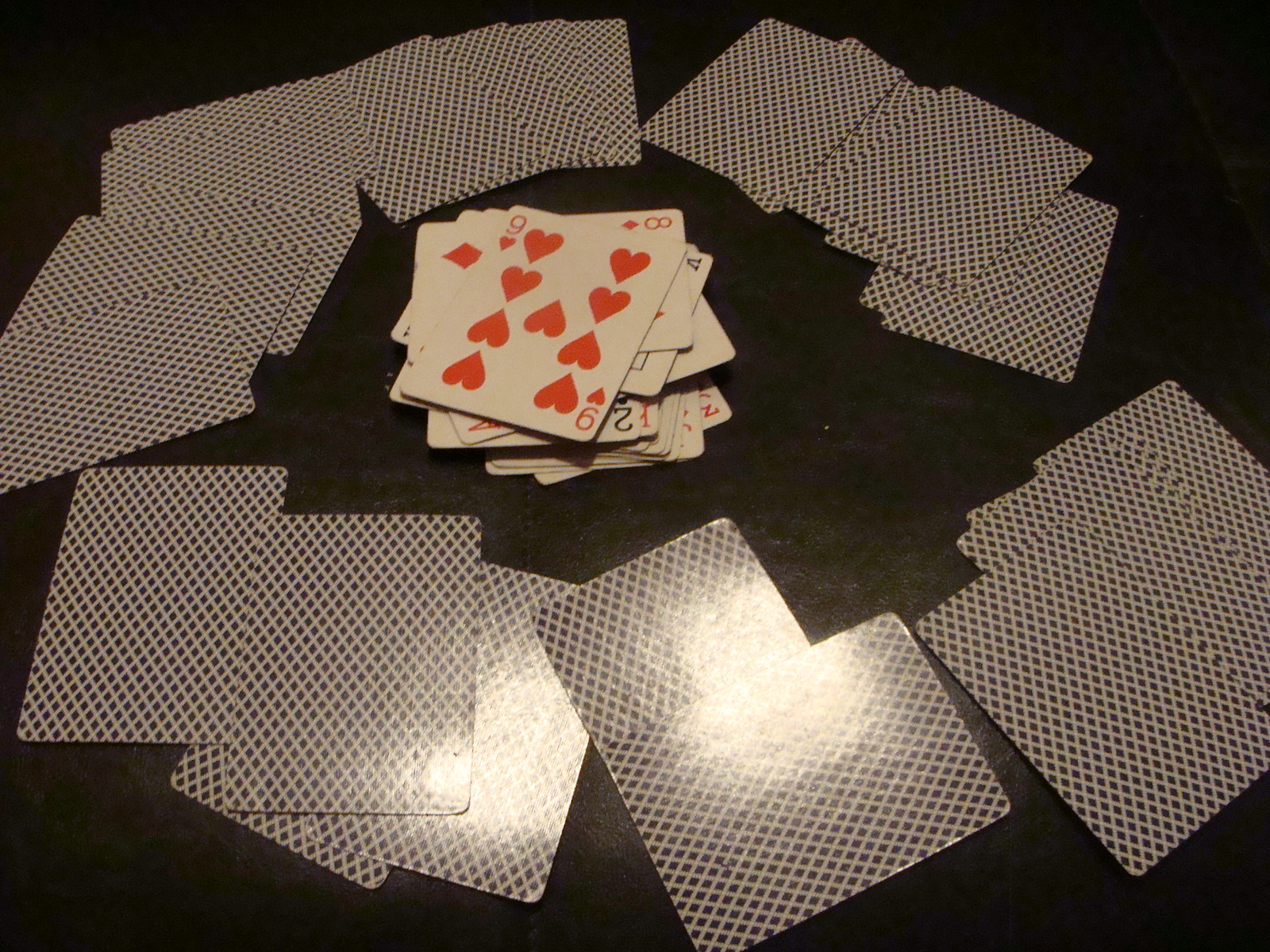A striking image featuring a black square as the backdrop sets a contrasting stage for a fan of white playing cards, which are meticulously arranged in a semi-circle. The stack of cards, totaling nine in number, includes the 9 of Hearts and the 8 of Diamonds, among others. Black dots are scattered across the cards, and a subtle light reflection adds a touch of brilliance to their pristine white surface. The arrangement is circular, although the cards do not meet at the center, creating an open, airy impression in the middle of the pattern.